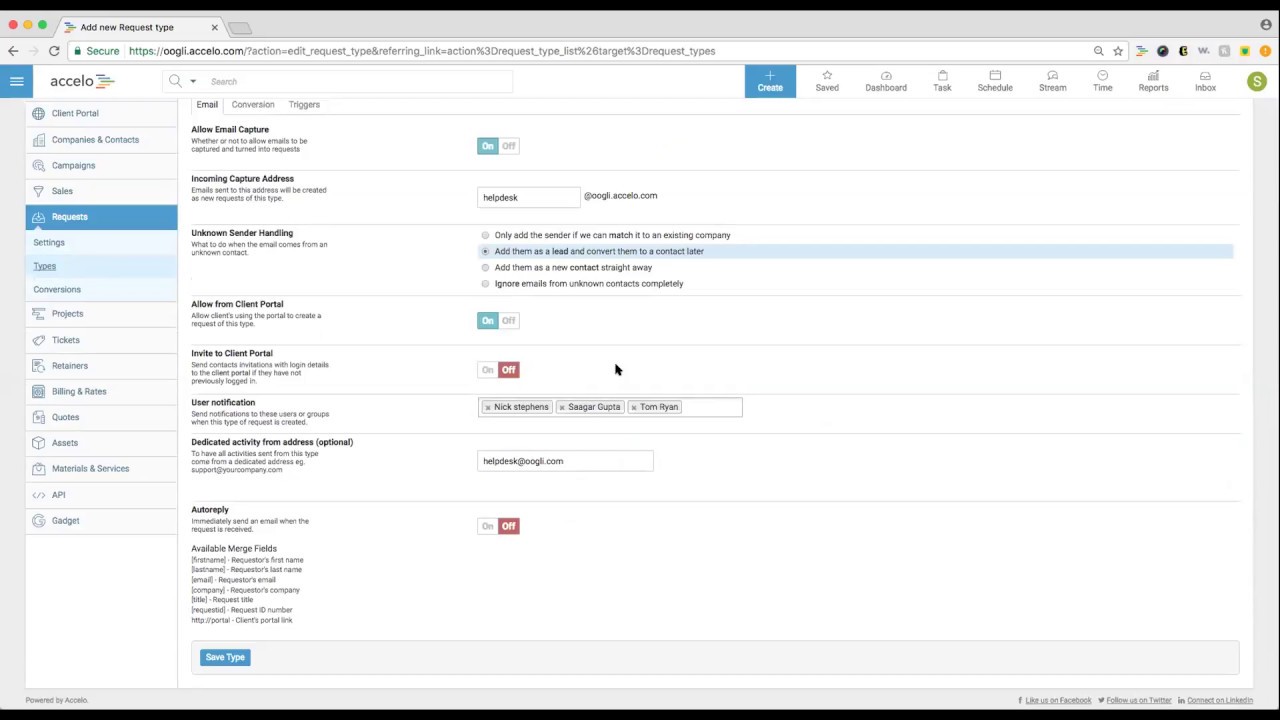The image is a detailed screenshot of what appears to be a complex software interface, possibly a management or data entry application. At the top, there are three primary icons in red, yellow, and blue aligned horizontally. Below these icons, there is a tab section resembling file tabs, featuring options such as "Add New" and "Request Type," along with a close button (X).

Adjacent to these tabs is a search bar, flanked by arrow icons on the left and additional icons on the right. To the left side of the interface, the word "Acelo" is prominently displayed, followed by a vertical list of approximately 15 items, each paired with its own tiny icon.

On the right side of the interface, eight distinct sections are present, each with headings in dark black text and subsections in lighter gray text. These sections include multiple on/off toggle switches, with at least one switch turned on (indicated by blue) and another turned off (indicated by red). Directly underneath these sections is another search bar, and a series of four brief entries accompanied by tiny icons, with the second entry highlighted in blue.

Further down, there is an additional on/off toggle switch that is in the 'on' position (blue), followed by another on/off toggle switch that is in the 'off' position (red). Below these switches are three more categorized sections, one more search box, and another red 'off' toggle switch. At the very bottom, there is a "Save Type" button.

Overall, the interface is packed with various interactive elements designed for detailed input and navigation, with a clear emphasis on organized categories and functional toggles.